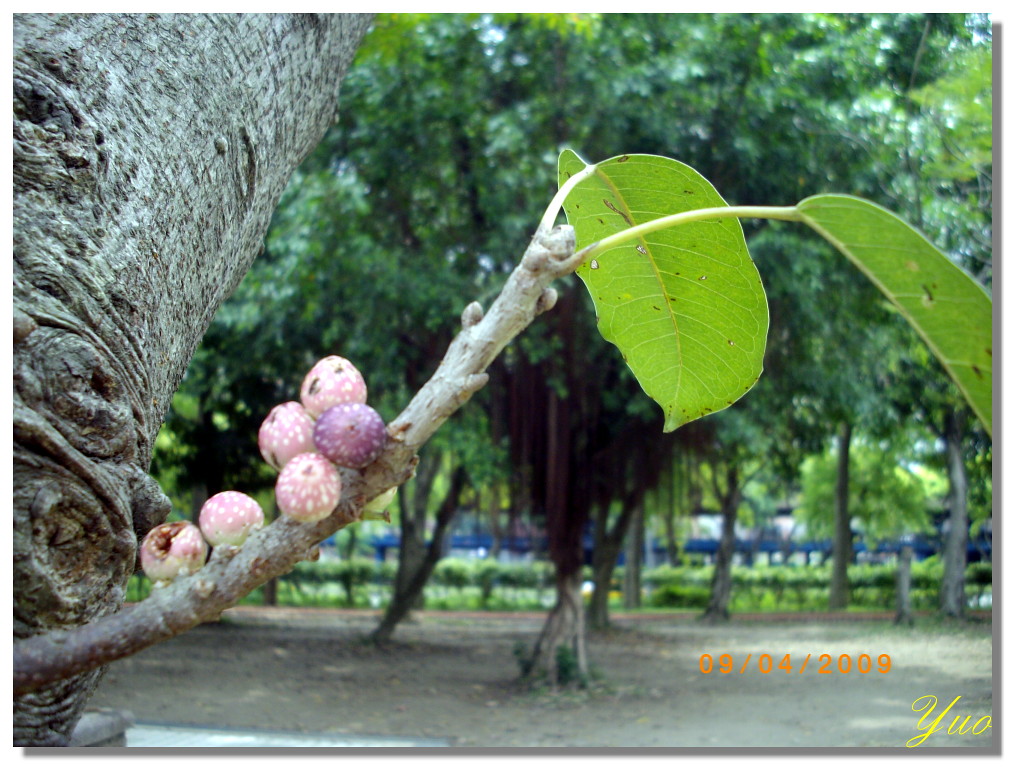The photograph is a clear, horizontal rectangular image prominently featuring a diagonal tree trunk on the left corner. Stretching out from the trunk is a single branch adorned with two leaves and clusters of small, round, purple or pinkish growths, possibly berries or nuts, numbering around six. The branch, in focus, contrasts against a slightly blurred background, enhancing its prominence. Behind this foreground, a wooden fence is visible, followed by a park-like area filled with more trees and greenery. The lower right corner of the image contains a watermark with the name "YUO" in yellow cursive script, slightly above which, in orange text, is the date "09/04/2009."